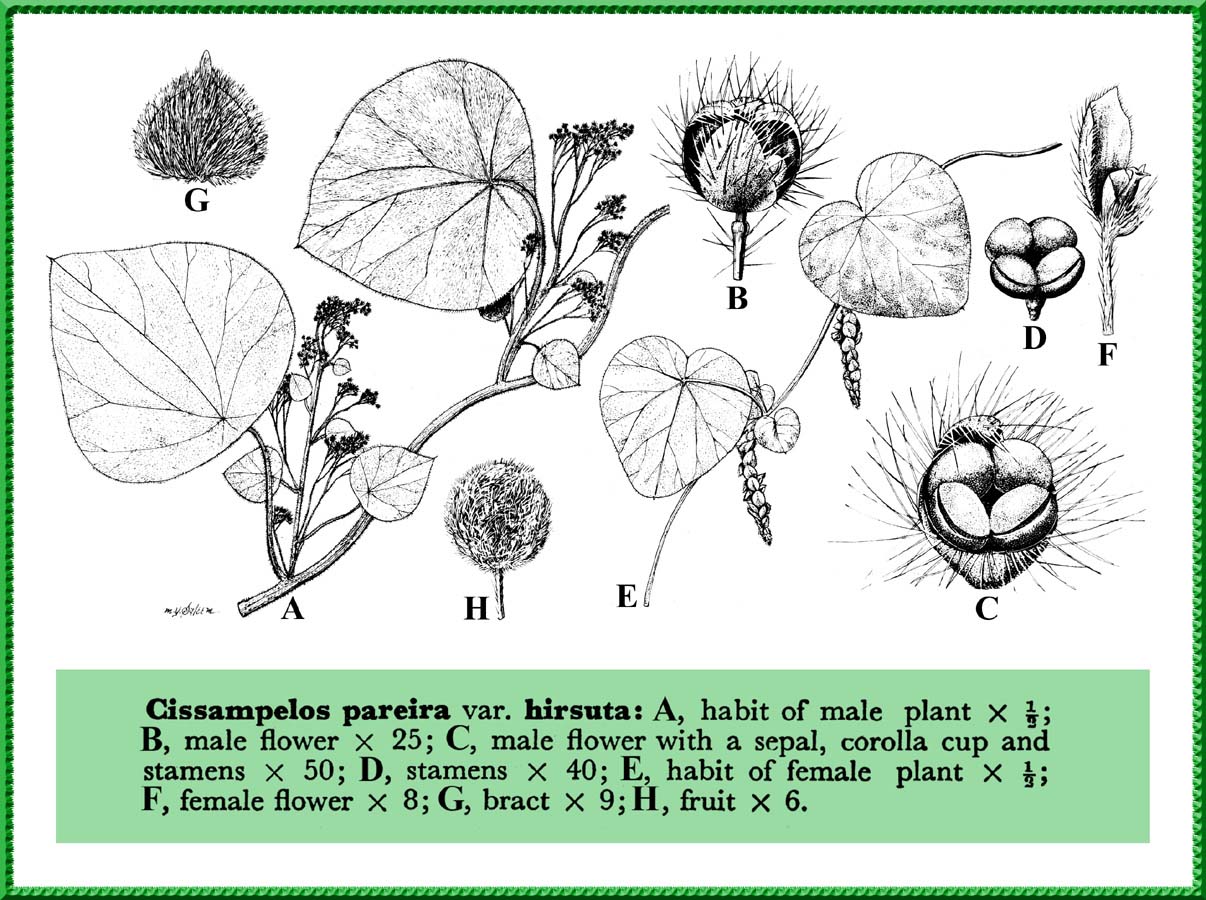This image is a detailed diagram of the Sysom Pallas Pyrrha plant, illustrating various parts labeled A through H. The background is a light green, transitioning to white in the upper section where black and white sketches of the plant parts are displayed. Each part of the plant, including some leaves and a piece of fruit, is meticulously labeled in black. The labels identify A as the habit of the male plant, B as the male flower, C as the male flower with a sepal, corolla, cup, and stamens, D as stamens, E as the habit of the female plant, F as the female flower, G as a bract, and H as the fruit. Below the illustrations, a green rectangle with black text provides the plant’s name: Sysom Pallas Pyrrha. Measurements of magnification are listed next to each label, though some are difficult to read. The border of the diagram has a green and black beaded appearance, adding a decorative touch to the scientific representation.